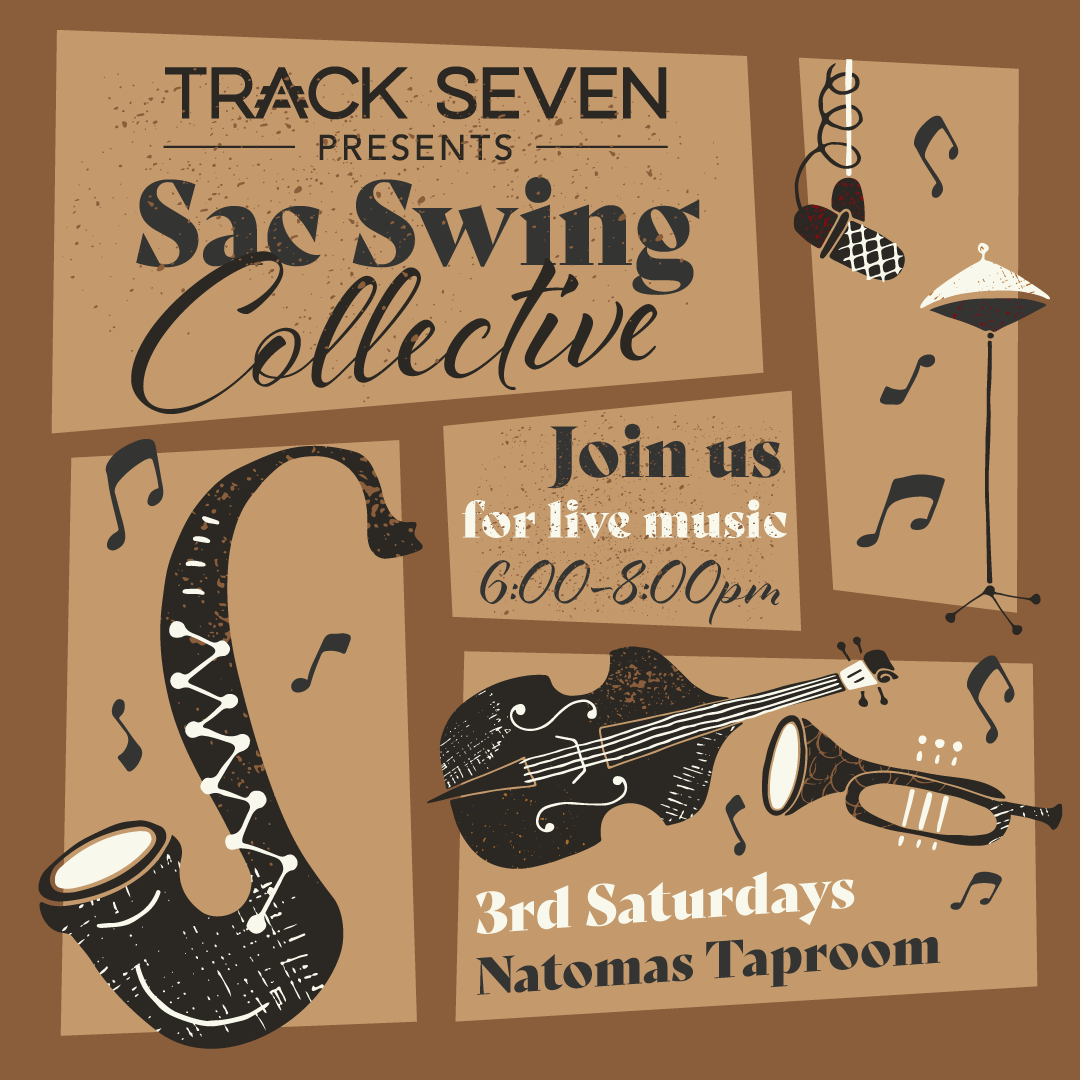The image is a digitized advertisement designed with a brown background and lighter brown blocks highlighting different sections. At the top left, the first block states "Track 7 presents Sax Swing Collective." Below this is a slightly longer block featuring illustrations of music notes, a microphone, and another instrument. In the center, there is a smaller block inviting viewers to "Join us for live music 6 to 8 p.m." On the left, another block shows a saxophone adorned with music notes in black and brown tones. The bottom right block reads "3rd Saturday Natomas Taproom," accompanied by images of a bass guitar, more music notes, and a horn. The writing is primarily in black, with some white, and the design includes modern depictions of various musical instruments like a saxophone, bass, trumpet, and cymbal.